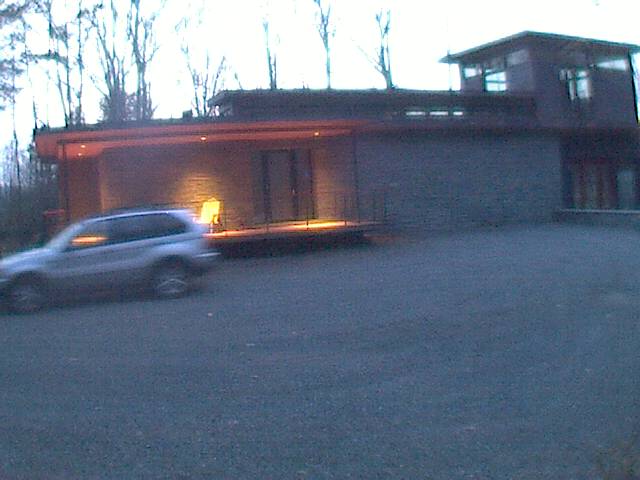A sleek silver car is driving towards the left, its wheels prominently visible. Behind the vehicle, an illuminated porch extends outward, featuring a ceiling and a railing. On the porch, a lone seat is positioned, appearing as though it’s casually placed there. The backdrop showcases a cluster of barren trees, their thin branches void of leaves, conveying a dormant state. The sky above is a stark white, adding a tranquil yet stark contrast to the scene. The surrounding wall is constructed from stone, giving it a robust, rustic appearance. On the left side, there is a door, while the top right section of the image reveals what seems to be an additional room, partially visible from the outside.